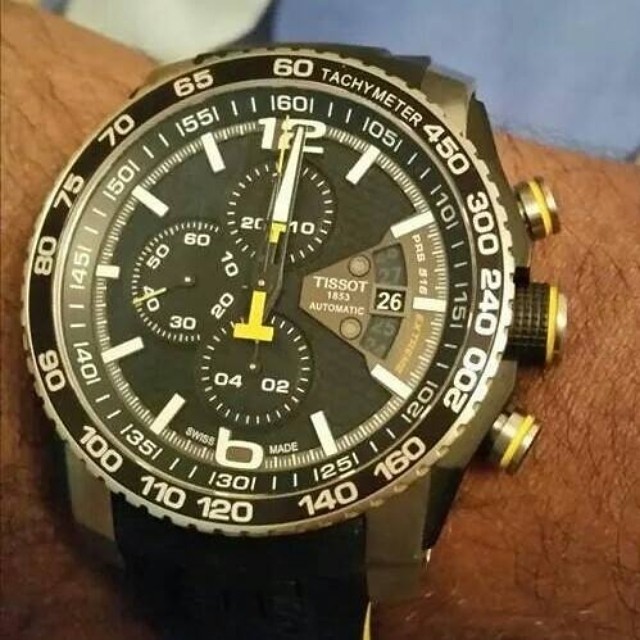In the image, there is a black coffee cup with a white interior set against a blue background. Adjacent to the cup, a man’s wrist is visible, adorned with an elegant watch. The watch features a black leather band and a silver casing. It is detailed with three buttons on its side, each featuring a unique design with silver and black hues encircled by yellow rings. The watch includes a tachometer on its outer edge, characterized by a black bezel and white numerical markings. The watch’s face is also black, showcasing numerals for the 12 and 6 positions, while the remaining hour markers are indicated by sleek white lines. The watch hands are white, complemented by a smaller yellow hand that stands out against the darker background. Additionally, the watch face is populated with various sub-dials and prominently displays the brand name "Ticot" along with the date indicator set at 26.